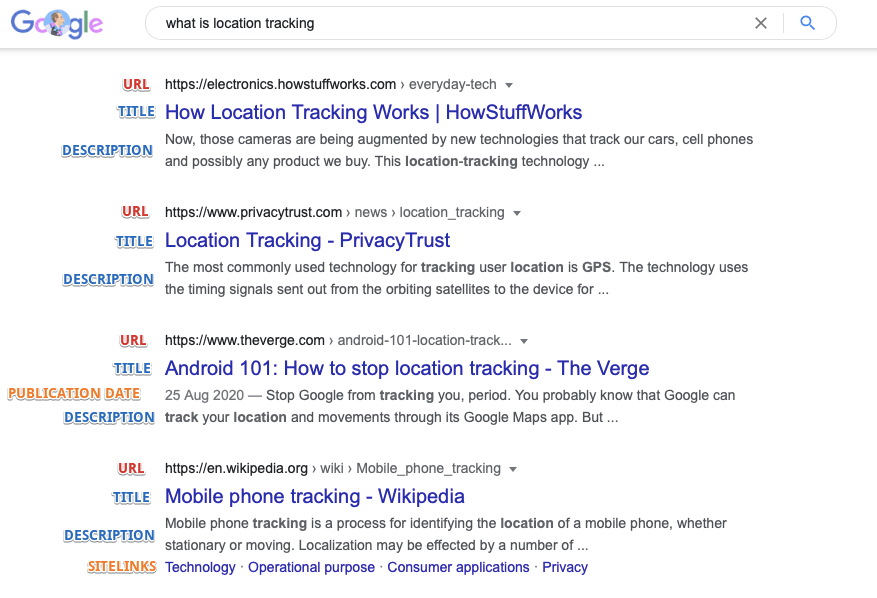In this image titled "What is Location Tracking?" displayed at the top, a Google search results page is shown with a search bar featuring colorful Google lettering in blue, purple, and pink hues. The search results below include four distinct entries, each annotated for clarity.

1. The first result is from the URL "electronics.howstuffworks." Its title is "How Location Tracking Works - HowStuffWorks" and the description reads, "Now those cameras are being augmented by new technologies; they track our car, cell phone, and possibly any product we buy." Annotations in red denote the URL, while the title and description are in blue.
  
2. The second result comes from "privacytrust.com" with the title "Location Tracking - Privacy Trust." The description is, "The most commonly used technology for tracking user location is GPS, which uses the timing signal sent from orbiting satellites." Again, the URL is marked in red with the title and description in blue.

3. The third entry is from "setveg.com" titled "Android 101: How to Stop Location Tracking." It is noted to be published on 25 August 2020. The description states, "Stop Google from tracking you. You probably know that Google can track your location and movement through its Google Maps app." The URL is in red, the title is blue, and both the description and publication date are black.

4. The final result is from "Wikipedia," titled "Mobile Tracking - Wikipedia." The description explains, "Mobile phone tracking is a process of identifying the location of a mobile phone whether stationary or moving." The site links are titled "Technology," "Operational Purposes," "Consumer Applications," and "Privacy." The annotations mark the URL in red, the title and site links in blue, while the description and publication date are in black.

This detailed breakdown includes color-coded annotations that effectively highlight each part of the search results, providing an educational snapshot of how location tracking information is presented in a Google search.